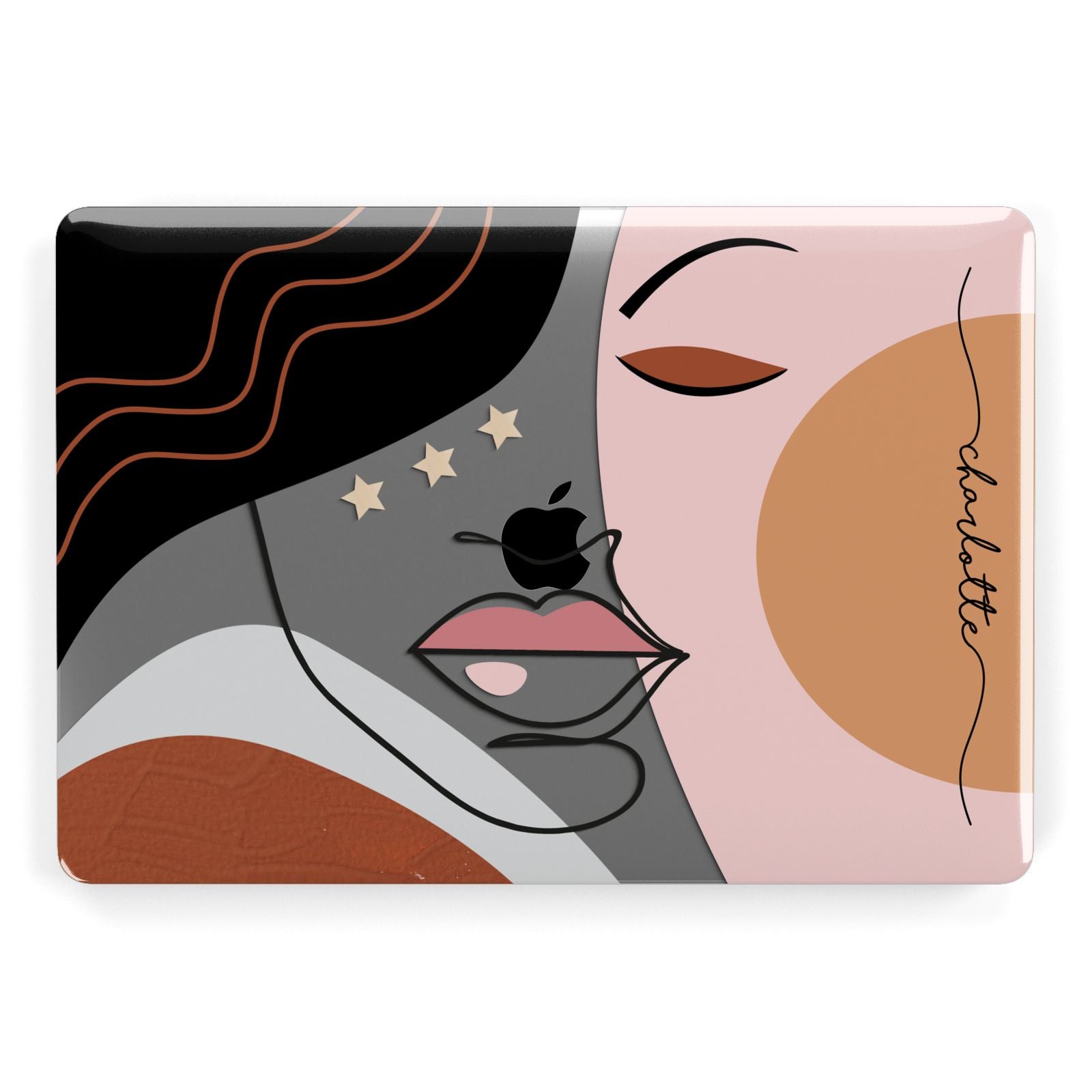The image is an abstract artwork displayed on what appears to be the cover of an Apple device, likely a tablet or laptop. Dominating the composition is a black Apple logo centered amidst the design. The artwork itself portrays a stylized, half-portrait of a woman's face. The face is rendered using a continuous black line that outlines features such as the chin, nose, and mouth, with various sections filled with vibrant colors.

A peach-pink tone fills the right side of the face, accentuating the woman's closed red eye and eyebrow. The lips are depicted with the upper part in pink and the lower part in gray. Above these features, an apple is positioned, suggesting her nose. The upper left corner of the image showcases a section of wavy black lines, presumably representing her hair. Orange squiggly lines cross this area, adding dynamic movement to the piece.

Additionally, three yellow stars can be seen alongside the face, enhancing the whimsical feel of the design. On the far right, a line of vertical text spells out "Charlotte," adding a personalized touch to the otherwise abstract interpretation.